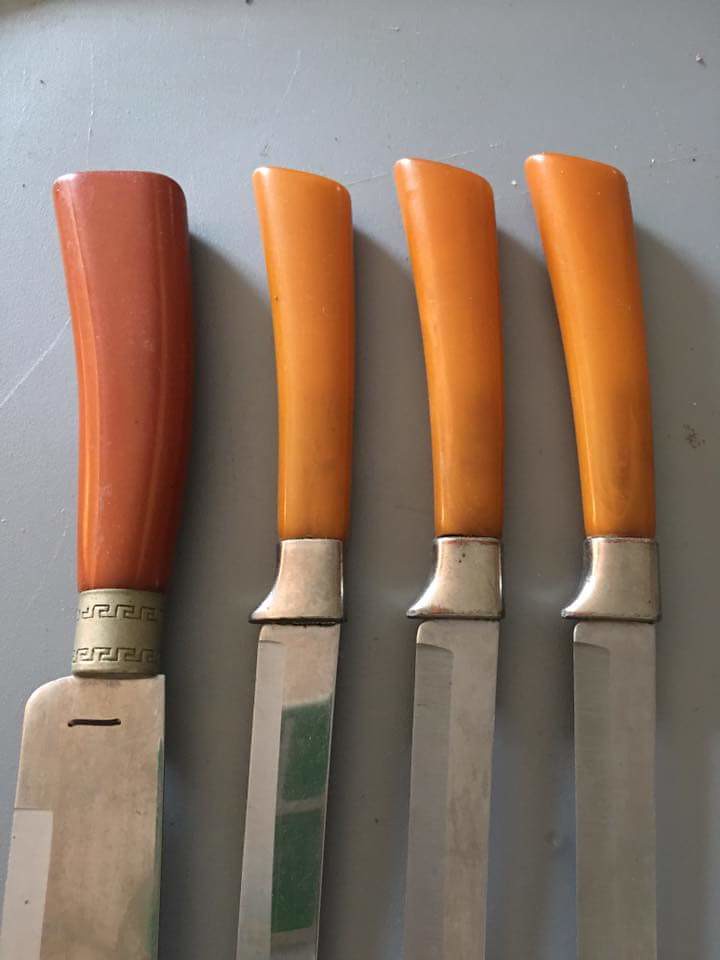In this close-up photograph, four knives are meticulously aligned vertically on a scratched, gray background, emphasizing both their handles and partial blades. The first knife, on the left, is notably larger and heftier, featuring a terracotta-colored, wooden handle that is thick and slightly curved, with an ornate metal bolster connecting the handle to its broad, rectangular blade. This knife stands apart, suggesting it might be a bread knife or a tool for heavier cutting. The other three knives, similarly old-fashioned in appearance, have matching light brown or peachy-orange, enamel handles with a gentle curve. Each of these smaller knives features a thin blade attached by a decorative silver piece, indicating they are likely part of a vintage dinner service set.